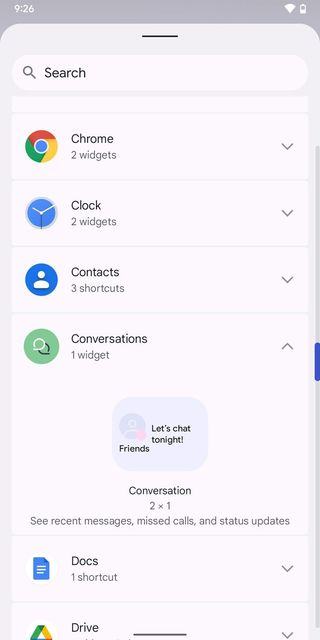A vertical smartphone screenshot is captured in this image, delineating various user interface elements against a backdrop of dark and medium gray gradients. At the top, a dark gray status bar presents the time "9:26 AM" on the upper left, with icons for Wi-Fi signal strength and battery level found on the upper right.

Below the status bar, the user interface of the device displays prominently. A search bar, identified by a magnifying glass icon, is positioned near the top center. Adjacent to this is the "Chrome" application icon along with the label "Chrome," followed by a series of text entries that read: "two widgets arrow down," "clock symbol, clock two widgets arrow down," and "context symbol, three shortcuts arrow down."

Proceeding further down, a green "Conversations" icon is visible, marked as "one widget arrow up." Below this, a chat dialog box displays the message "Let's chat tonight, friends" in black text. A description underneath reads: "Two times one, see recent messages, missed calls, and status updates."

Finally, at the bottom portion of the image, there are icons representing docks and a drive, each accompanied by a respective arrow indicating possible further interaction or navigation options.